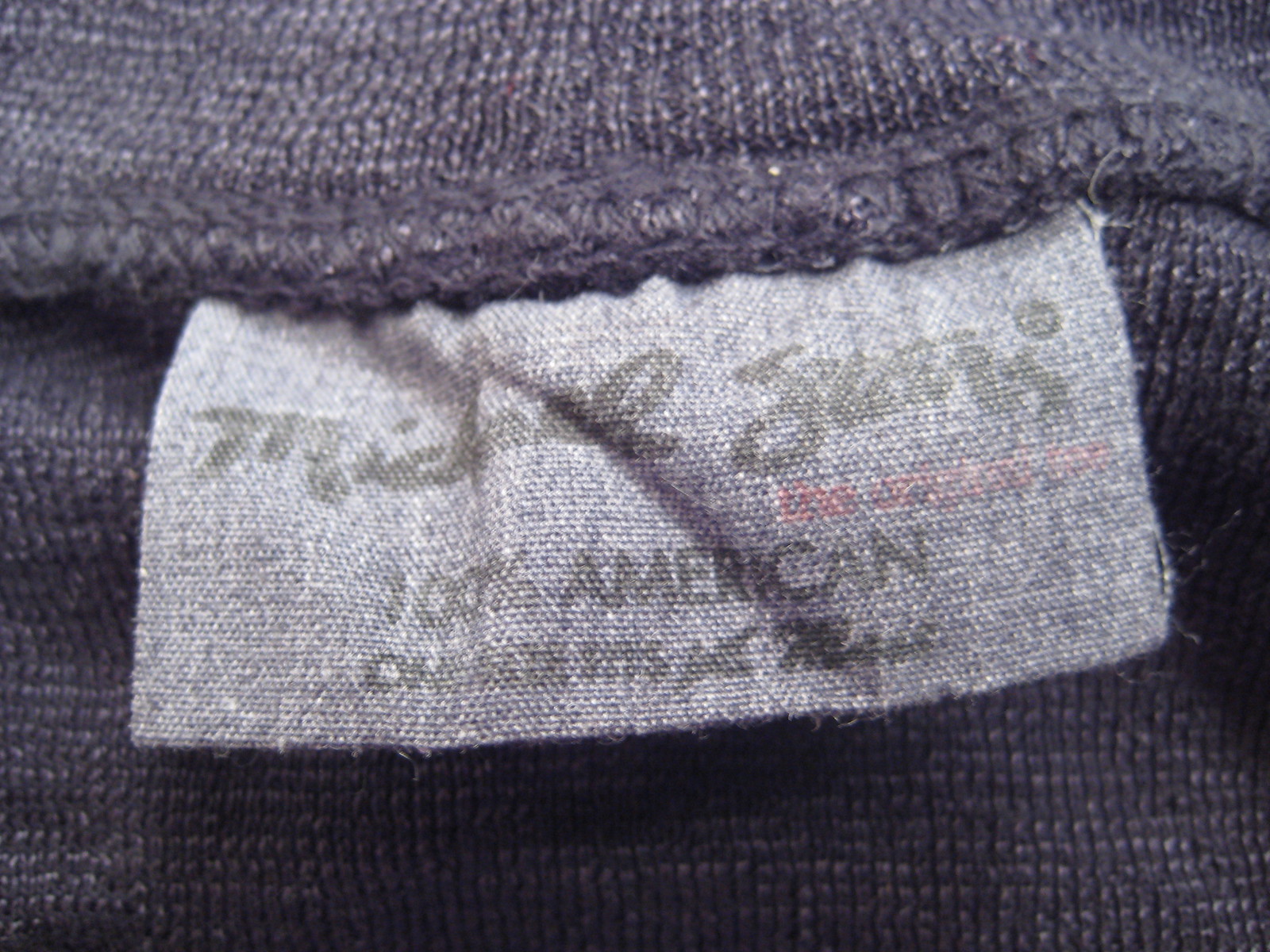A close-up of a clothing label sewn into the seam of a garment. The fabric of the garment is a dark navy blue with specks of white, giving it a textured appearance. The stitching along the seam appears to be machine-sewn. The label itself is a faded light grey or light blue denim, making some of the text difficult to read. The visible portion of the label displays the brand name "Michael" on the left-hand side, though part of the brand name is obscured. Below the brand name, the text reads "100% American."